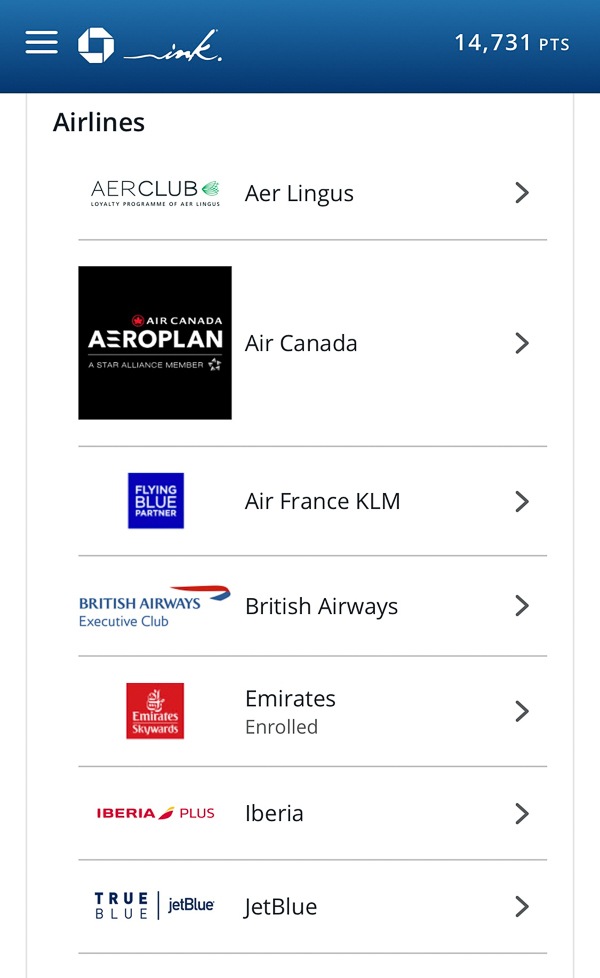The image displays the Chase, Inc. app user interface, showcasing a detailed view of the points and airline partners section. In the upper right corner, the user has accumulated 14,731 points. On the upper left, there's a hamburger menu icon for navigation. The top of the screen features the Chase, Inc. logo, with "Inc." written in a cursive lowercase font to the right of the Chase icon, which consists of four interlocking panels surrounding a blank square.

Below this header, there's a tab labeled "Airlines." Listed under this tab are various airline loyalty programs:

1. **AER Club** — AER Lingus.
2. **Air Canada Aeroplan** — An option accompanied by the Air Canada logo.
3. **Flying Blue Partner** — Identified by a blue icon, representing Air France KLM.
4. **British Airways Executive Club** — Pertaining to British Airways.
5. **Emirates Skywards** — Displayed with a red logo and white text, indicating the user is enrolled.
6. **Iberia Plus** — For Iberia Airlines.
7. **True Blue JetBlue** — For JetBlue Airlines.

Each program option is separated by thin grey lines. A one-pixel grey border runs vertically along the right and left edges of the list. Additionally, there are small grey two-sided arrows on the right side of each option panel. The background of the interface is white, and the bottom navigation menu buttons are not visible in the image.